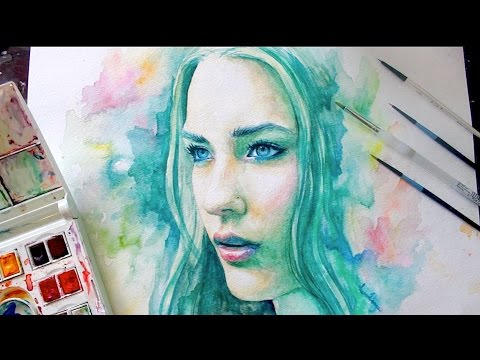This image captures a screenshot from a video showcasing a watercolor painting in progress. The painting, set against a black background with black bars at the top and bottom indicating a video format, features a detailed, realistic portrait of a woman's face. The woman's hair, depicted in aquas, blues, and greens, suggests a blonde hue beneath the artistic colors. Her expressive blue eyes gaze wistfully off to the left, framed by a cloud-like mix of watercolors in pink, yellow, and green that seamlessly blend with her hair. Her lips are slightly parted, adding to the pensive expression.

To the bottom left of the shot, a well-used watercolor palette is visible, showing remnants of various colors—predominantly yellow, green, black, reddish hues, and bits of blue. Off to the right, resting on the canvas, are four watercolor brushes, two smaller and two larger, appearing momentarily unused. The entire setup shows the meticulous process and intricate details involved in creating this vibrant watercolor portrait.